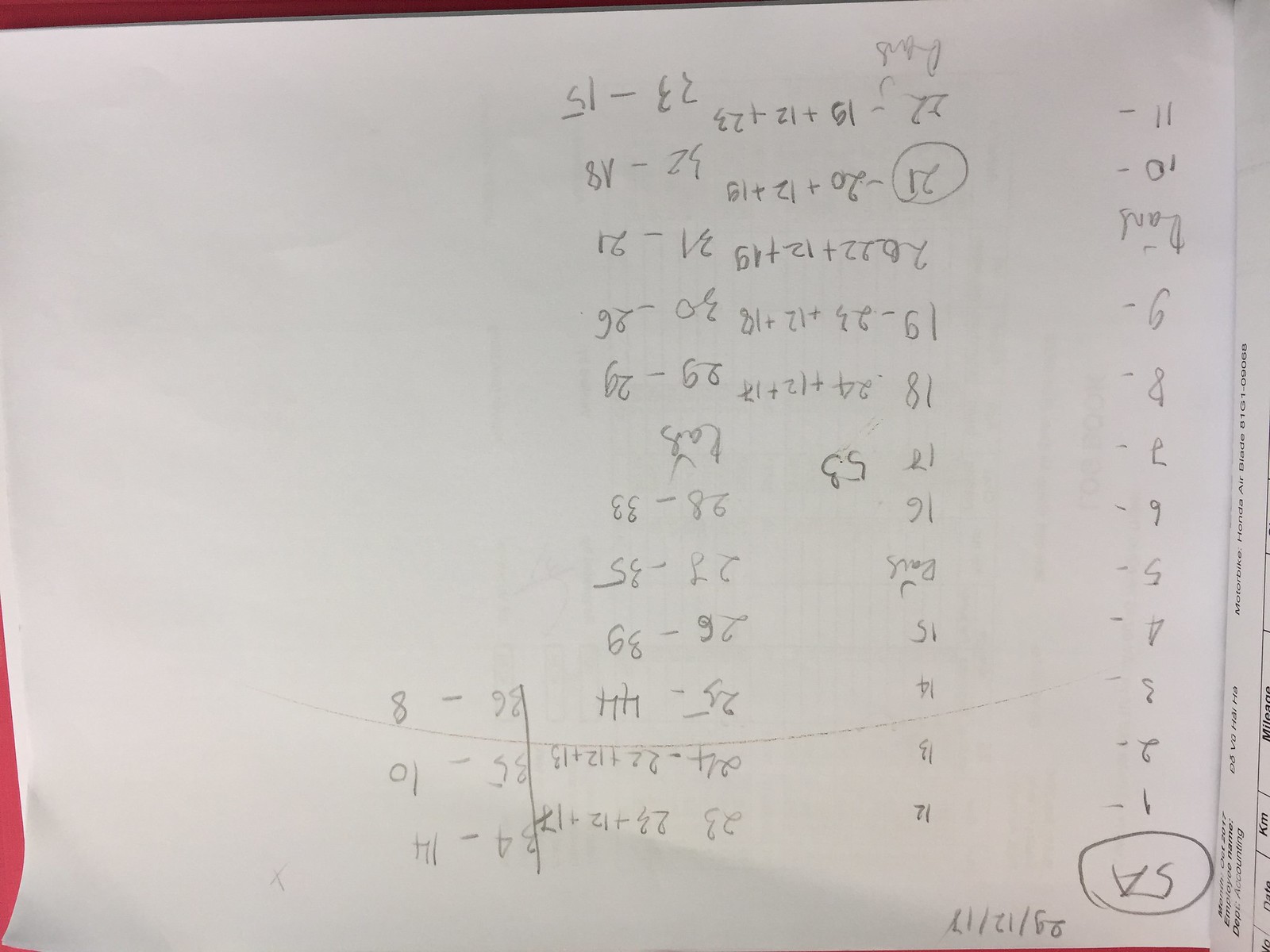This photograph showcases a mathematics homework assignment written in average handwriting, oriented upside-down. The assignment features a series of sequentially numbered lines, starting with -1 and progressing through 1, 2, 3, 4, 5, 6, 7, 8, 9, skipping a line, and then continuing with 10 and 11. Each line is filled with mathematical expressions involving addition and subtraction. There is an additional line with text between numbers 9 and 10, creating a total of 12 lines. Toward the top left corner of the image, above the list of numbers, there is a partially legible date—specifically the digits "1218". The text and calculations appear to have been part of a workbook or assignment page. Overall, this image presents the intricate details of a mathematics exercise, framed in a somewhat chaotic manner due to its upside-down orientation.